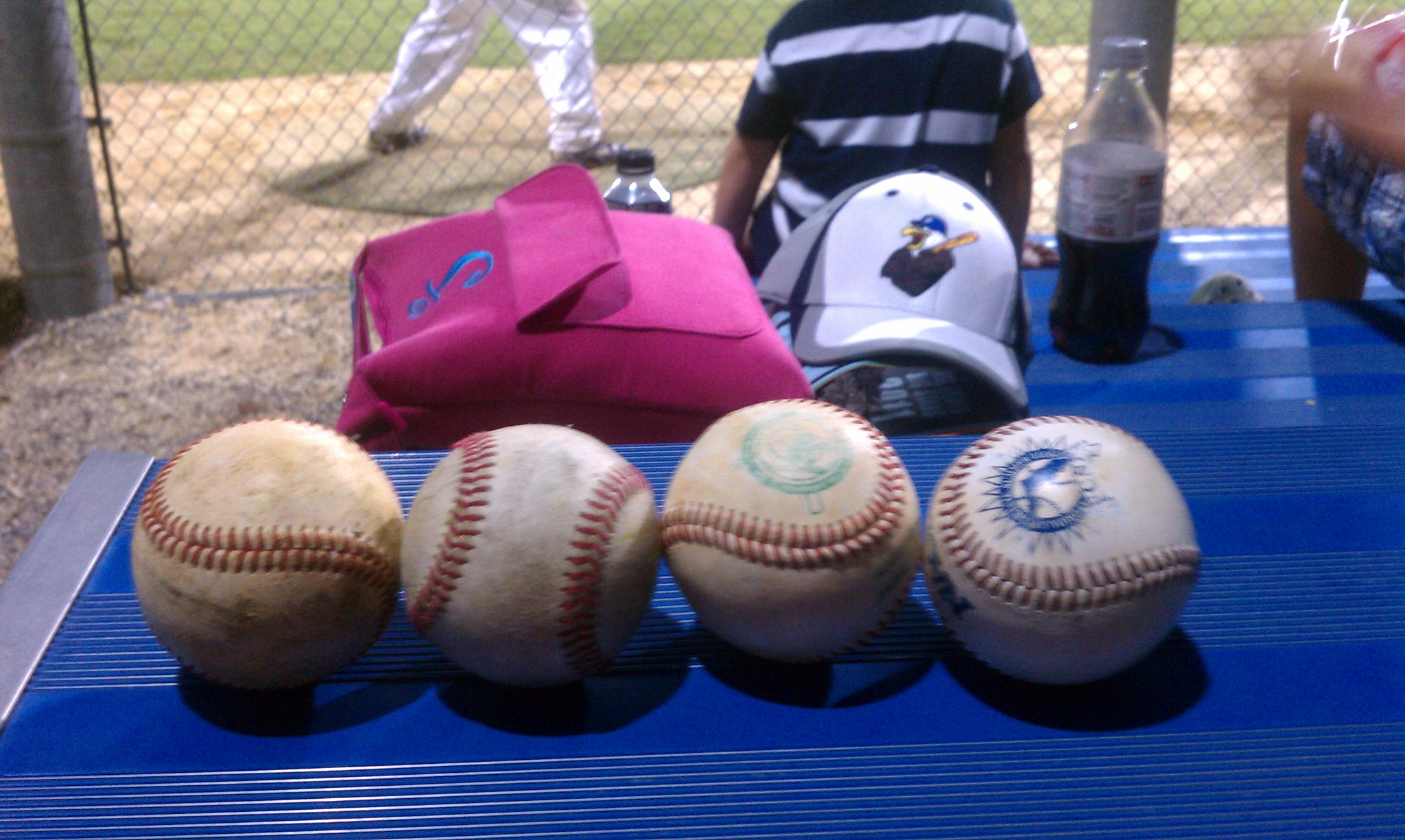This detailed image captures a vibrant scene at a baseball event. In the foreground on a blue bleacher, four baseballs lay side by side in a row, each with distinct characteristics: two are noticeably dirty, one has a green symbol, and another bears a blue symbol. All the balls feature prominent red arch stitching. To the left of the balls sits a pink backpack with a blue symbol on it, juxtaposed by a white cap adorned with a cartoon eagle wearing a blue cap. Nearby, a mix of beverages includes bottles of soda and crystal juice. Pivoting to the middle of the frame, a person in white pants stands on a mound, likely a pitcher given their stance, surrounded by sandy dirt and green grass. Behind them, another individual in a black shirt with white stripes sits on a blue bench, hands planted on the edge, observing the scene through a chain-link fence. To the right, another observer is partially visible, clad in a dress. The sunlight casts distinct shadows, adding depth to this bustling baseball tableau.